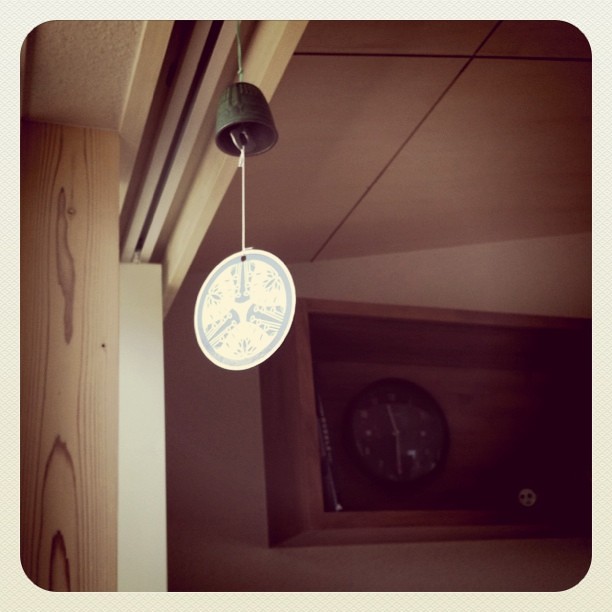A photograph captures the scene within a doorway, showcasing a decorative wind chime prominently. The wind chime features a green fabric string suspending a matching green cup-shaped bell. Inside the bell, a metal hook supports a white string that culminates in a blue and white ornate, lace-like circle. In the background, the ceiling and walls are painted a warm tan color. Adjacent to the doorway, a dark brown cabinet with a shelf is visible, holding a book and a clock. The door frame is crafted from light-colored wood, and beside it, a white slide track indicates the presence of a sliding door.